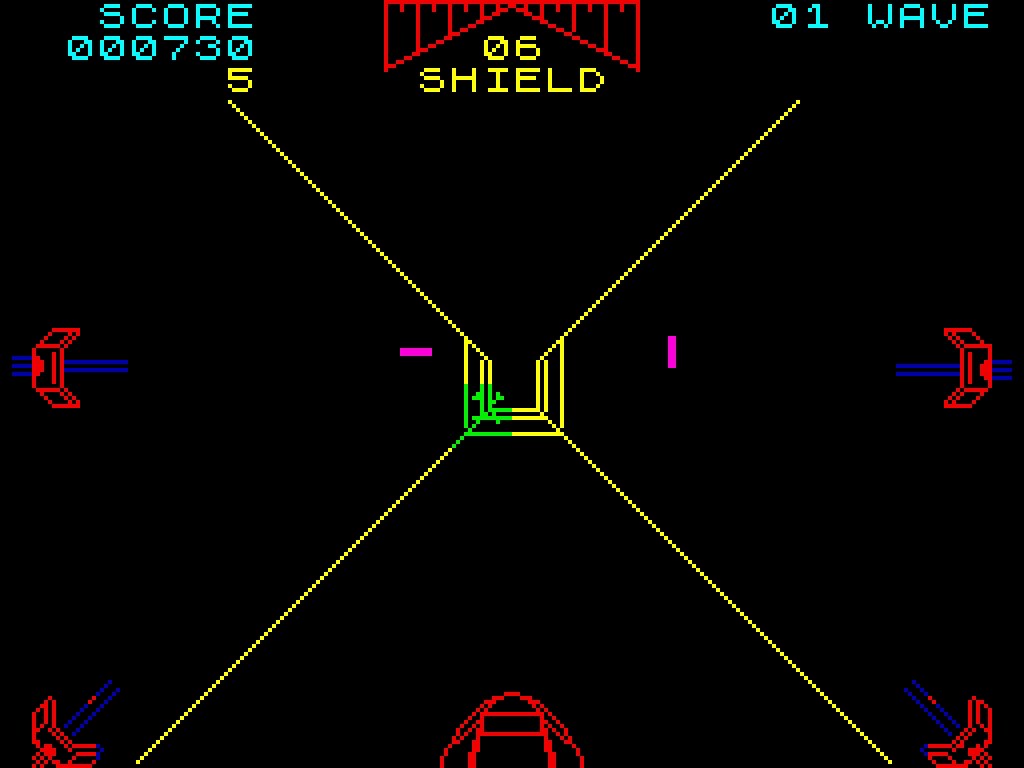The image is a screen capture from a minimalist video game with a predominantly black background. In the upper left corner, teal-colored text displays the score as "000730." Dominating the center of the screen is a red, angled structure that evokes the appearance of a ruler, with its bottom section rising towards the center. Directly beneath this structure, yellow text reads "06 SHIELD." 

In the upper right corner, more teal text states "01 WAVE." The main focal point of the image is a thin X-shaped object with an open-top box in the center. Flanking this X shape to the left and right are two rudimentary red ships. Each ship features two horizontal blue lines extending inward, pointing towards the center of the screen. The overall visual is stark and geometric, emphasizing simplicity and retro aesthetics.